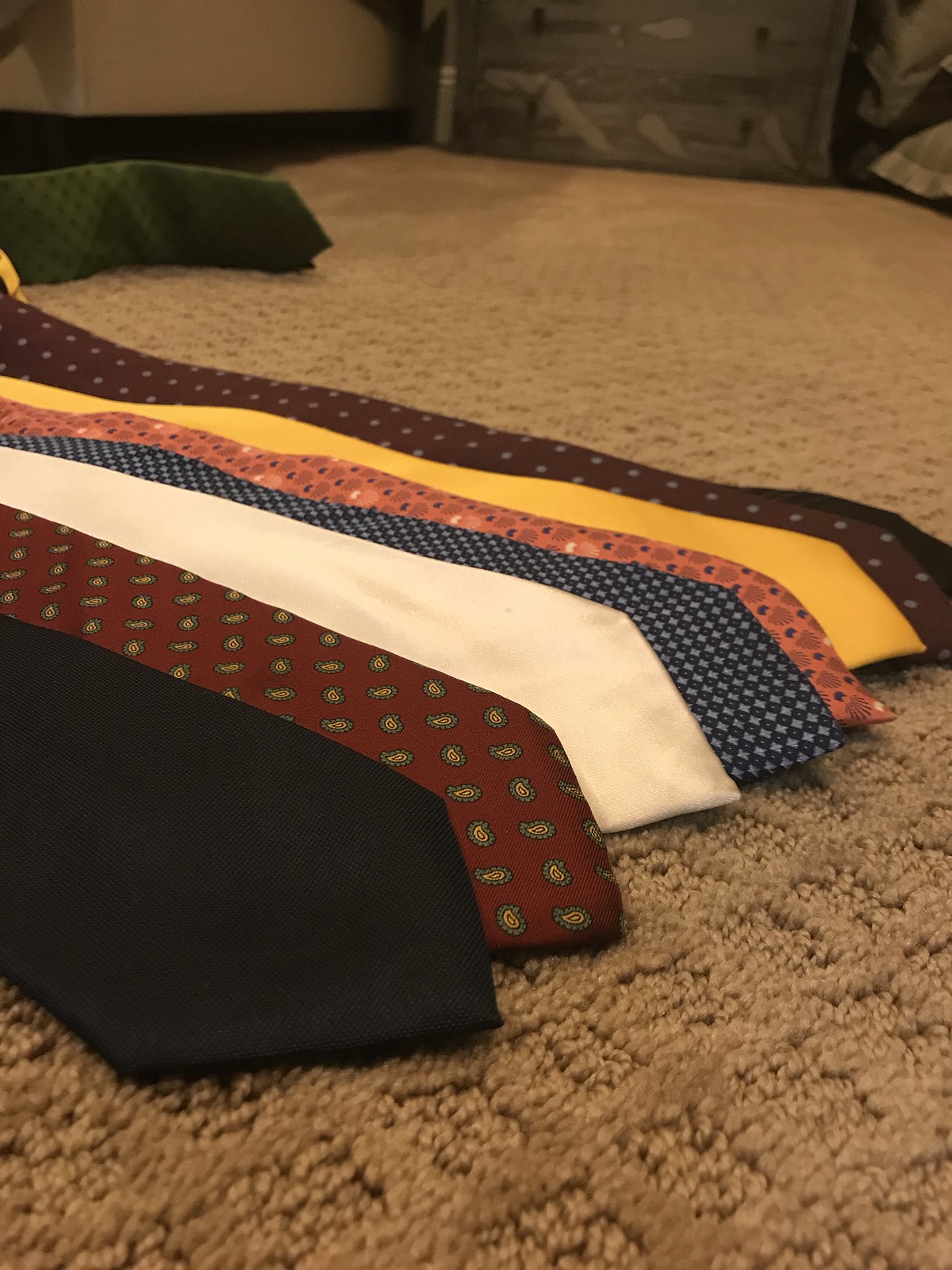In this detailed image, a series of neckties is meticulously arranged on a carpeted floor. The photograph captures a close-up view from a low angle, emphasizing primarily the bottom halves of the ties, which are positioned in a slightly overlapping manner along an angled line. The beige carpet features an intricate honeycomb texture, subtly visible beneath the ties. 

There are at least seven ties visible in the foreground, each showcasing a unique design and color palette. The first tie, closest to the camera, is solid black. Following it is a red tie adorned with a green potato-like pattern. The third tie is completely white, while the fourth features a dark blue and light blue checkered pattern. Next is a tie displaying a pinkish-orange hue with black and light gray heart designs. The sixth tie is a solid yellow, and the seventh appears to be a dark red or burgundy with a similar potato pattern as the second tie.

In the background, partially visible, is a dark green pillow that rests on the carpet, further contributing to the rich texture of the scene. The arrangements and designs of the ties, paired with the detailed texture of the carpet, create a visually compelling tableau.